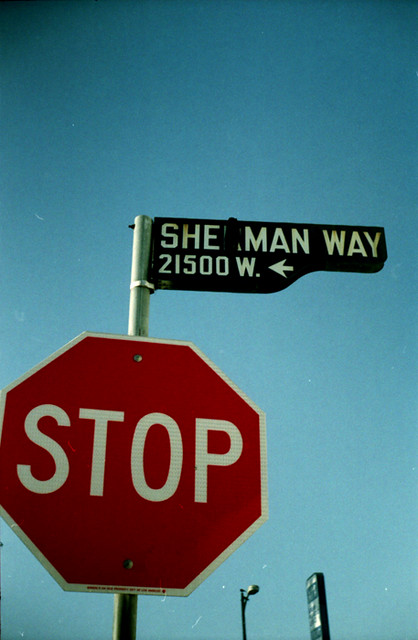In this image, we observe an upward perspective of a standard stop sign mounted on a greenish-colored pole. The stop sign itself is hexagonal with white outer lines, distinctively red in color, with the word "STOP" prominently displayed in the center in white letters. Above the stop sign, there is a black sign with white lettering that reads "SHE," with a crossed-out letter, followed by "M-A-N-WAY." Further down the same pole, there is yet another sign displaying "21500 W." with a white arrow pointing to the left. Also visible are the top portion of a light post and an additional sign. The entire scene is set against a gradient blue background that is lighter at the bottom and gradually darkens towards the top.